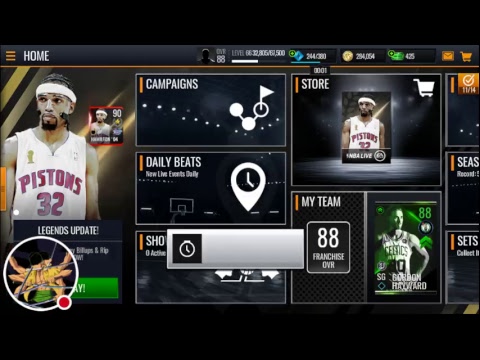This screenshot captures a basketball video game interface. At the top of the screen, there is a menu button labeled "Home," followed by the player's profile icon, which is currently a blank, faceless image. The profile displays "OVR 88" indicating the overall rating, and "Level 66." It also shows some numerical values, possibly progress toward the next milestone, represented as "32805 / 450500." Beneath these details, there is an experience bar showing the player's progress.

To the right, three types of in-game currency are displayed: a blue diamond-shaped currency with a current total of 244 out of 380, a gold circle-shaped currency totaling 294,054, and a green rectangular currency amounting to 425. Adjacent to these currencies are an orange email button and an orange shopping cart icon.

The main portion of the screen features images of a basketball player wearing a Pistons number 32 jersey. Surrounding the images are windows for various game modes and features, including Campaigns, Daily Beats, My Team, Store, Legends Update, Seasons, Sets, and Shows.

Additionally, there is a semi-transparent pop-up in the center of the screen, represented as a blank silver rectangle with the image of a stopwatch, possibly indicating a timed event or notification.